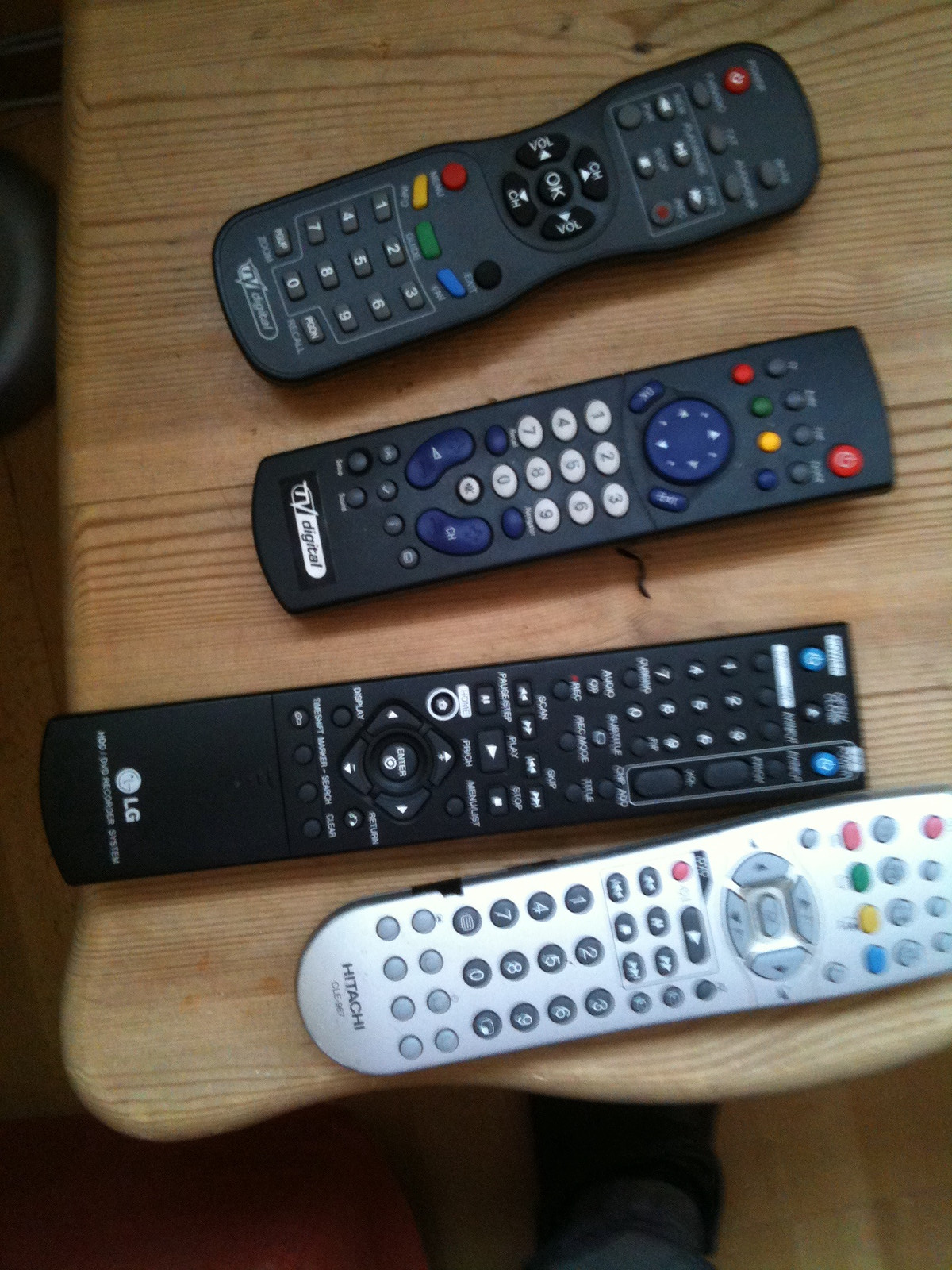A photo taken from above shows four remote controls placed horizontally across a light beige wooden table with wavy edges, likely a maple surface. The remotes are lined up with their bottoms on the left and tops on the right, partially cutting off the first and last remotes from view. Starting from the bottom, the lowest remote is silver, curved at the bottom, and sports the brand name "Hitachi" on the left side in black lettering. This remote has numerous buttons, likely around twenty. Just above it is a black LG remote, long and thin, featuring both white and blue buttons. The third remote, still black but lighter in shade, has the words "TV Digital" written on it, with a mix of white and colorful buttons—red, blue, green, and yellow. The final remote at the top also says "TV Digital" but comes in a slightly different style with gray and black buttons. Additionally, part of the photographer's leg and foot can be seen in the bottom right-hand corner of the image, along with a dark brown floor area adjacent to the table.